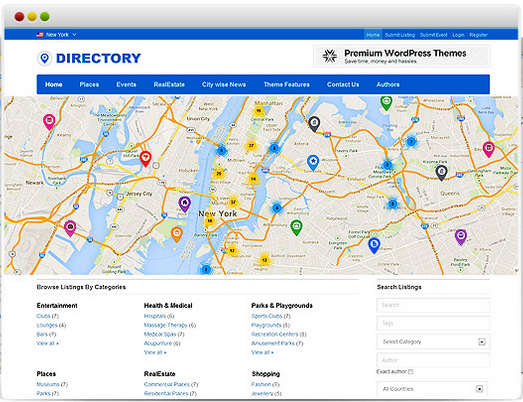In this detailed image, we observe a directory page designed for listing various categories and events. At the top right, the text "Premium WordPress Themes" emphasizes the advantages of saving time, money, and avoiding hassles. On the top left, the site is identified with the word "Directory" written in blue. Positioned above this on a blue header, "New York" is prominently displayed, indicating the regional focus of the directory. Moving to the far right of the header, functional buttons including "Home," "Submit Listing," "Submit Event," "Login," and "Register" are present for user navigation.

Beneath the header, we encounter a secondary white header featuring the directory title alongside the recognizable WordPress logo. This section also houses navigation buttons for "Home," "Places," "Events," "Real Estate," "City," "Wise News," "Theme Features," "Contact Us," and "Authors," ensuring comprehensive site exploration.

Dominating the central part of the image is a detailed map, vividly marked with various colored pins and points of interest representing the geographical areas of New York and New Jersey. Below this visual display, a white section categorizes multiple listings under the heading "Browse Listings by Categories." This section breaks down into specific categories such as Entertainment, Places, Health and Medical, Real Estate, Parks and Playgrounds, and Shopping, each accompanied by further subcategories for more refined browsing.